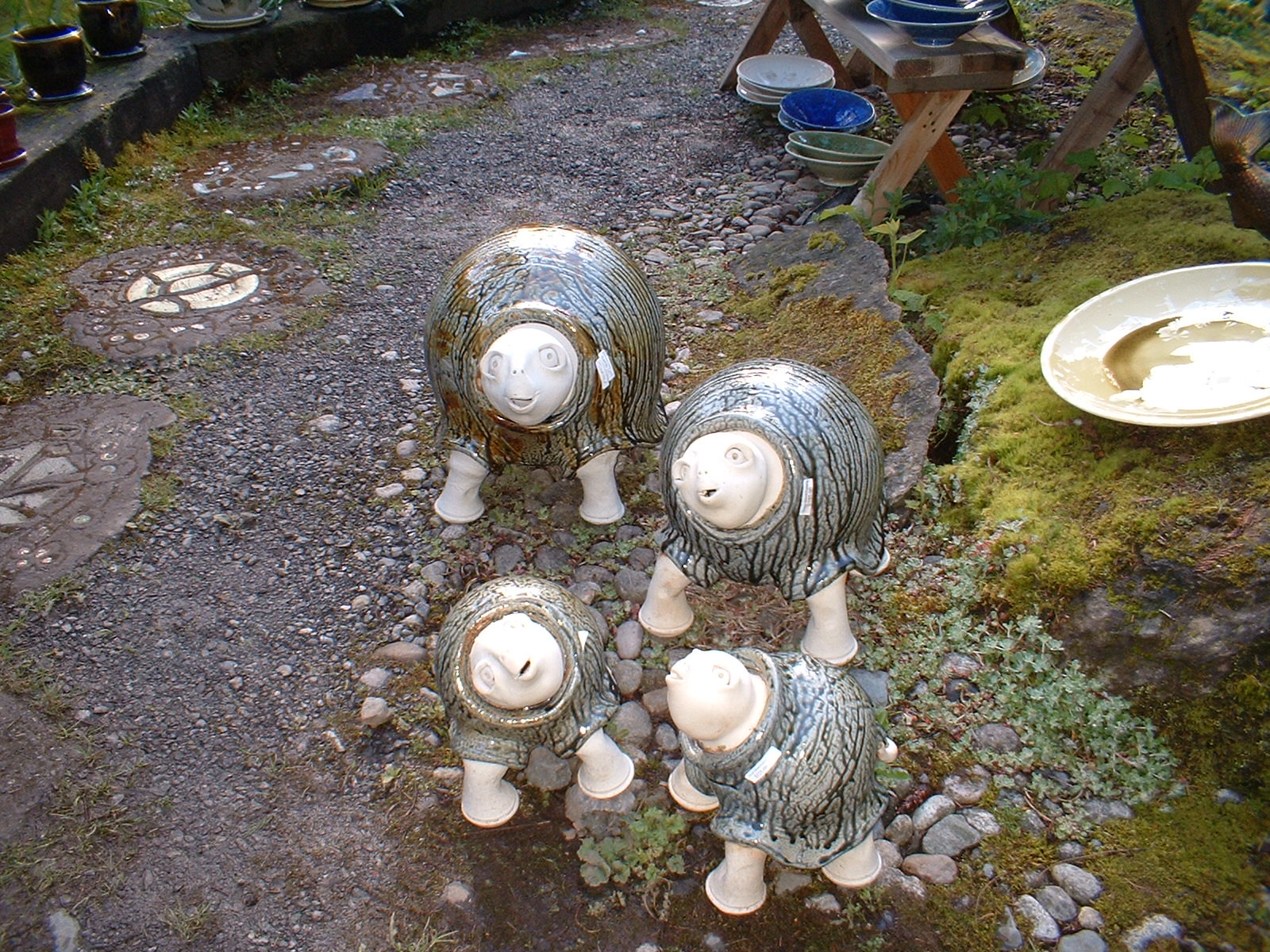The image captures a garden scene with four ceramic garden decorations that resemble whimsical turtle-like creatures, each encased in glossy, marble-striped shells. They are positioned on a gravel and dirt surface, surrounded by patches of grass. The angle suggests the photo was taken from a slightly elevated position, providing a clear view of the creatures and their surroundings. To the side of the figures, there is a rustic wooden table adorned with various dishes and vases, hinting at a possible ceramic sales area. Additionally, a plate with dirty water and a small puddle can be seen near the creatures. Their rounded bodies and large, expressive eyes make them appear lively and endearing, with one figure looking straight ahead, another turning its head, a third standing on its back legs, and the fourth glancing back. The scene evokes a quaint, artistic ambiance with a touch of nature's charm.